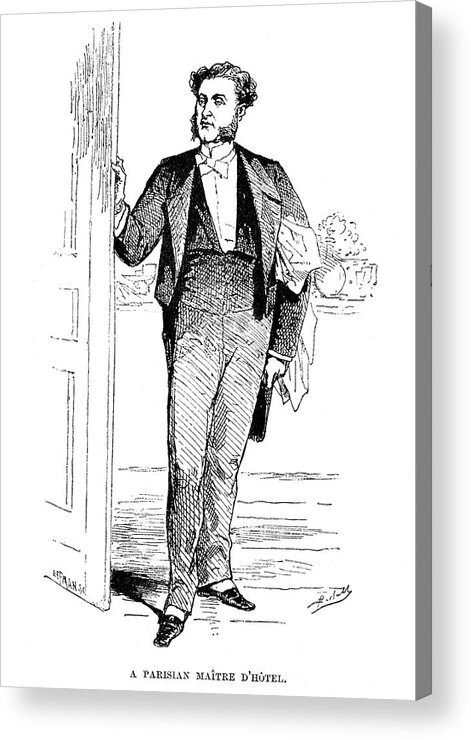A highly detailed pencil-style illustration, possibly a print from a vintage book, captures a serene yet enigmatic moment. The drawing portrays a Parisian maître d'hôtel, impeccably dressed in a formal suit complete with a waistcoat and pointed shoes. With pronounced sideburns and bouffant, bushy hair, the man stands at the threshold of a door, delicately pushing it open with his right hand, while his left hand rests at his side. His face bears an inquisitive yet melancholic expression as he gazes into the house. 

Behind him, a faintly sketched garden scene softly blurs the boundary between indoor and outdoor spaces, providing a subdued backdrop to the detailed foreground. The image is rendered on a white background, but intriguingly, it includes a three-dimensional grey side, suggesting that the illustration is presented on a three-dimensional canvas or object rather than a flat sheet of paper. Annotated at the bottom with the label "a Parisian maître d'hôtel," the image captures both the formality and subtle poignancy of its subject.